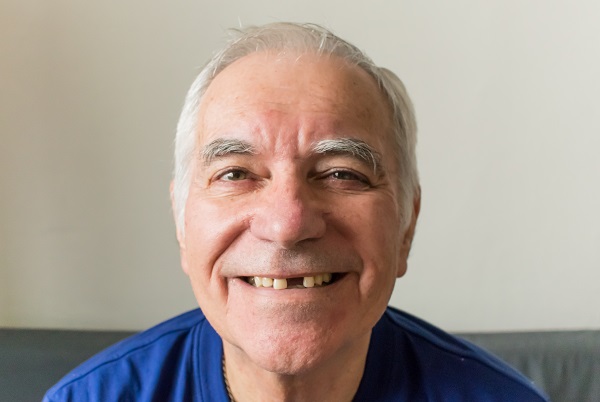In this color photograph, we see an elderly man, likely in his 70s or early 80s, smiling warmly at the camera. He has a receding hairline with greyish white hair and bushy, thick eyebrows that feature a mix of grey and white strands. His light-colored skin is illuminated by his broad smile, which reveals a missing front tooth on the left side of his face. The man is dressed in a royal blue crew neck shirt, with a glimpse of a chain visible on the right side of his neck. He appears to be seated on a grey sofa, which spans the width of the image in the background, set against a light grey wall. The photograph, captured in a landscape orientation with a realistic style, focuses on the man’s facial features and joyful expression, emphasizing a sense of warmth and character.